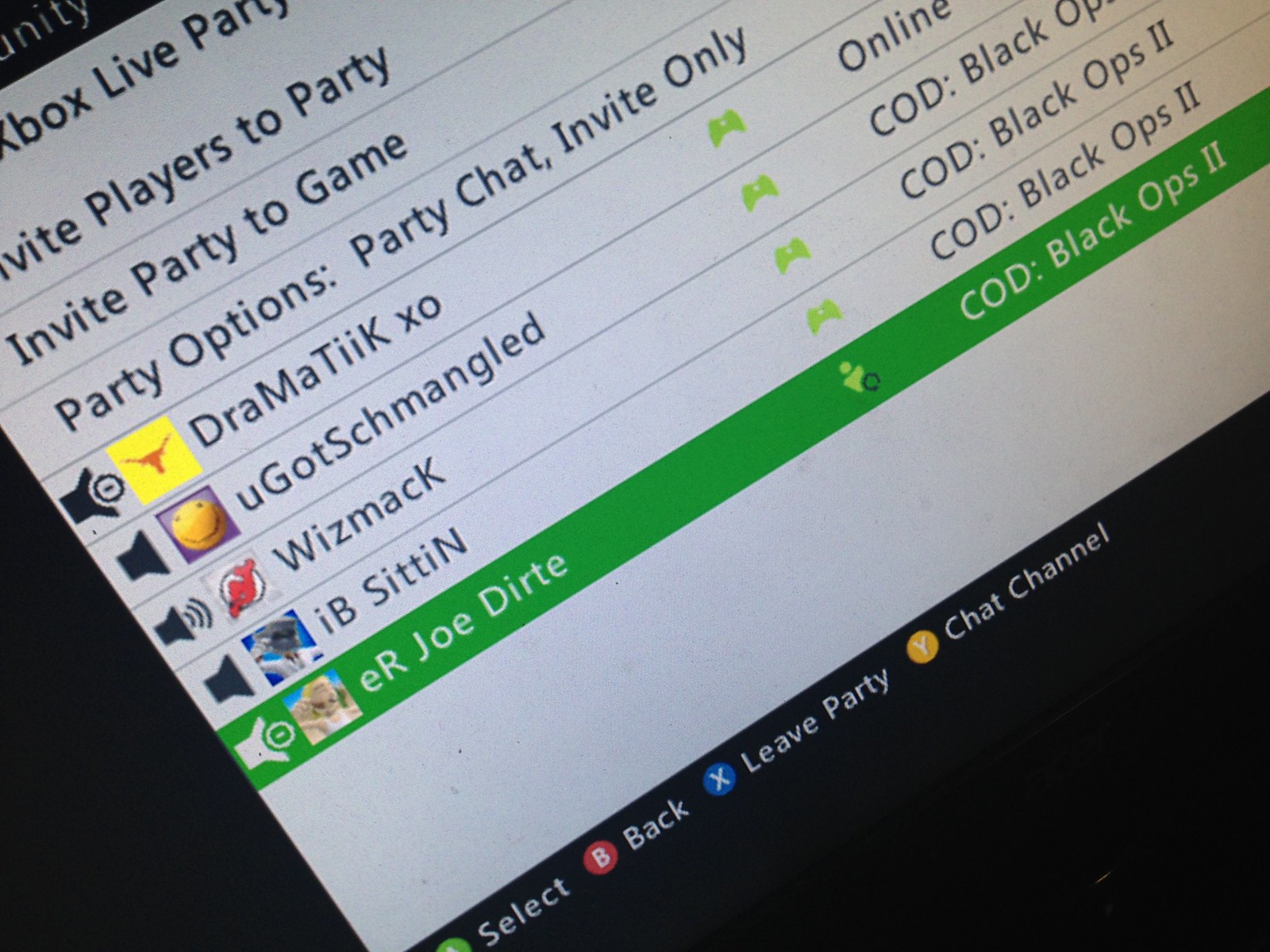The photograph shows a slightly tilted screen displaying an "Xbox Live Party" interface. At the top, it features options like "invite players to party," "invite party to game," "party options," "party chat," and "invite only." The image quality and angle cut off some text, making it hard to see perfectly. The lower part of the screen has colored buttons labeled: the green button for selecting, the red button for going back, the blue 'X' button for leaving the party, and the yellow 'Y' button for the chat channel. Five players are visibly listed; the first is online, while the next four are associated with "COD Black Ops 2," indicating their participation in the Call of Duty: Black Ops 2 game. The most colorful section highlights a user (possibly named Joe Dirt or E) active in the game. The photograph suggests an invitation setup for gamers to join a session.